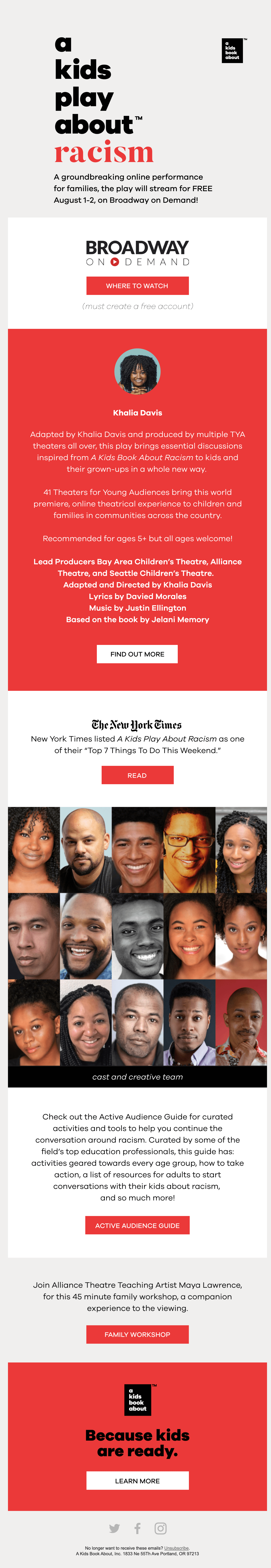In this highly compressed and somewhat illegible screenshot, the main focus is on an announcement for an online event titled “A Kid’s Play About Racism.” The heading features black text for “a kid’s play about” and the word “racism” prominently highlighted in red. Below the title, a brief but impactful description reads, “A groundbreaking online performance for families. The play will stream for free August 1st through 2nd on Broadway On Demand.” 

Further down, the platform “Broadway On Demand” is mentioned again, followed by a slightly unreadable, smushed-together description about Kalia Davis. Next, it is highlighted that “The New York Times” has rated “A Kid’s Play About Racism” as one of their top seven things to do this weekend.

Accompanying this information is a grid of 15 photographs, featuring individuals who are either smiling or looking directly at the camera, each presumably involved in the performance. Lastly, the screenshot includes a series of red rectangle buttons, which likely function as interactive links or call-to-action prompts for the viewer.